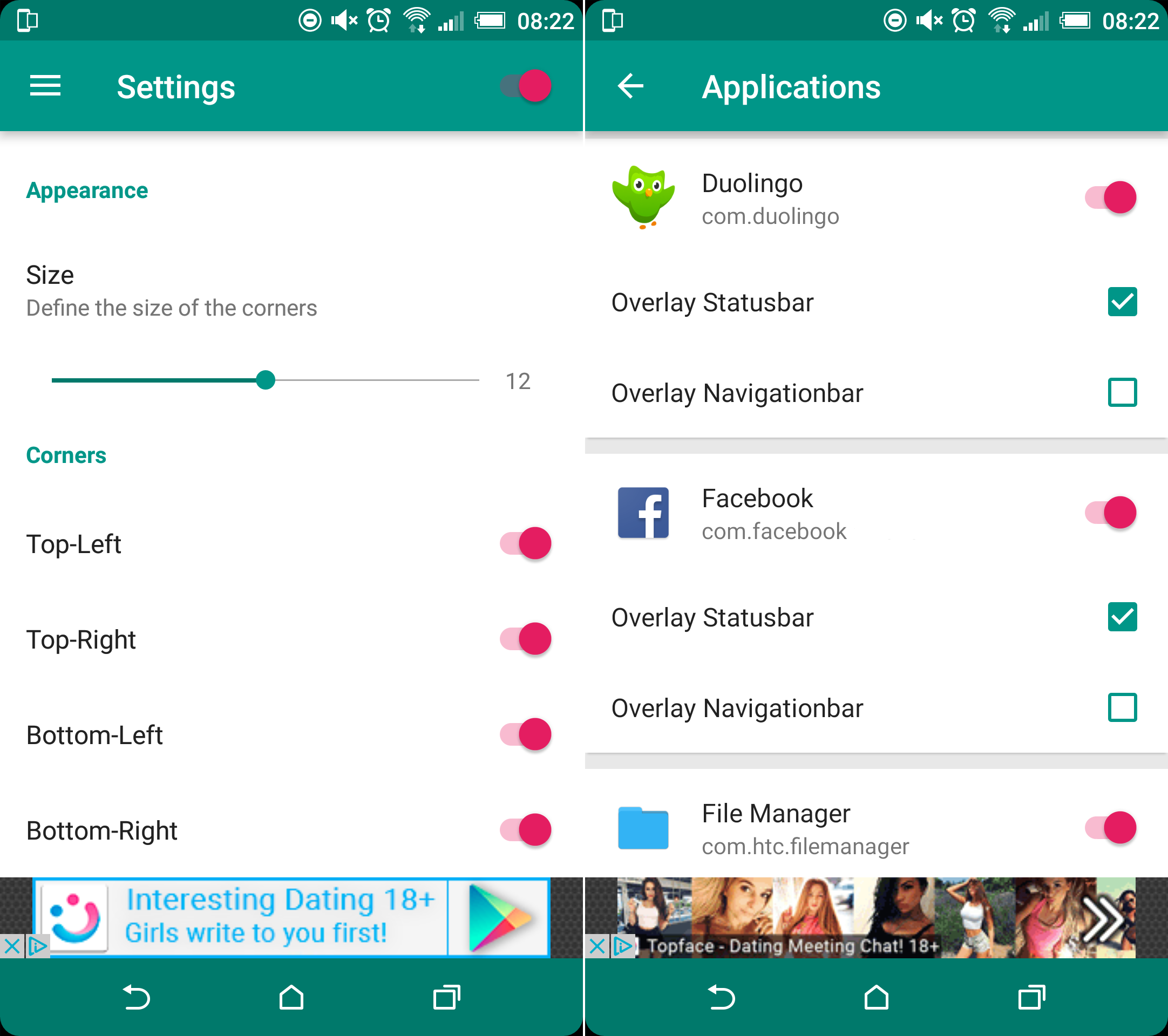The image consists of two detailed screenshots of an Android phone's application interface.

**Left Screenshot:**
- The status bar at the top displays standard phone icons.
- The central section shows a "Settings" menu, highlighted in green.
- Directly below "Settings" is a category labeled "Appearance."
- Within "Appearance," there is a sub-option titled "Size," with text explaining it allows the user to "define the size of the corners," which is currently set to 12.
- The "Corners" section lists adjustable options for "Top Left," "Top Right," "Bottom Left," and "Bottom Right," each accompanied by red icons.
- Toward the bottom, there is an advertisement for an 18+ dating site, featuring the text "Interesting dating 18+, girls write to you first."

**Right Screenshot:**
- The top section displays the "Applications" menu.
- Listed applications include "Duolingo," marked with its recognizable owl character and a red icon.
  - The entry for Duolingo has a checked option for "Overlay status bar" and an unchecked option for "Overlay navigation bar."
- "Facebook" is next, identified by its icon and also paired with a red icon.
  - Facebook similarly has "Overlay status bar" checked and "Overlay navigation bar" unchecked.
- "File Manager" follows, marked by a blue file icon and a red icon.
  - Below File Manager bears the same check and uncheck pattern.
- Another advertisement appears at the bottom for "Top Face," a dating app for users 18 and up, displaying photos of different women.

Overall, the screenshots illustrate various settings and application adjustments on an Android device, interspersed with dating app advertisements.